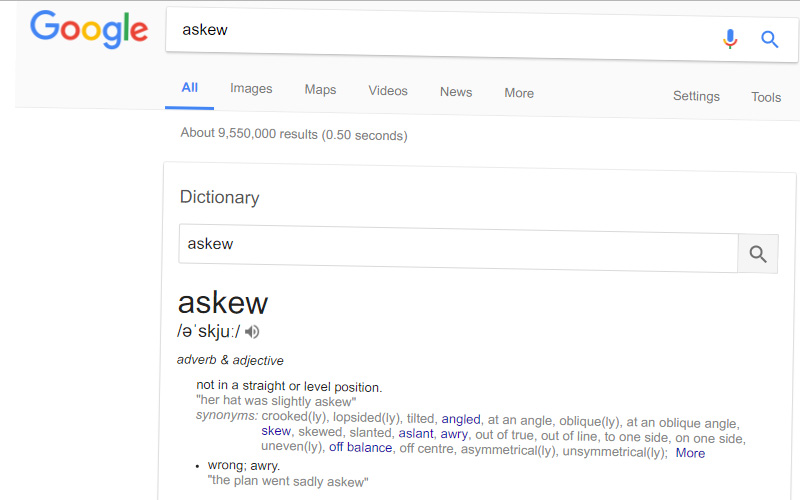This screenshot captures a page of Google search results for the term "ASKU". The Google logo is prominently displayed at the top left, adjacent to the search box containing "ASKU". The search box features both a microphone icon and a magnifying glass icon. Below the search bar, the word "ALL" is highlighted in blue, indicating the current tab, alongside other options such as Images, Maps, Videos, News, More, Settings, and Tools. 

The page reports approximately 9,550,000 results found in 0.50 seconds. The default result section is a dictionary entry for "ASKU". This entry repeats the search term "ASKU" and includes an audio pronunciation icon. The term is defined as an adverb and adjective meaning "not in a straight or level position", with an example usage: "Her hat was slightly askew". Various synonyms are listed, such as crookedly, lopsidedly, tilted, angled, and others. Further usage and related words include terms like wrong, awry, planar, and another mention of "slightly askew".